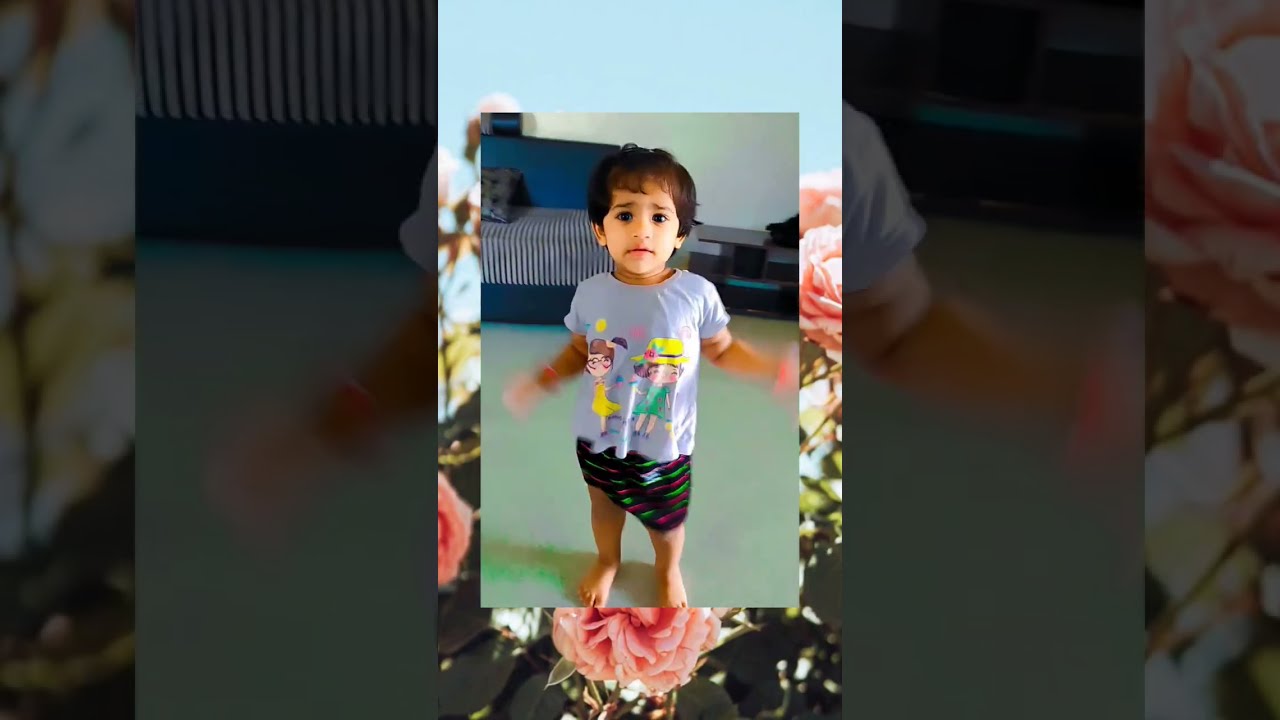In this image, a little boy of around three to four years old stands barefoot in a living room, appearing somewhat distressed or worried. He has big brown eyes and dark hair. He is wearing black shorts with diagonal pink and green stripes and a blue short-sleeve shirt featuring two cartoon characters—a girl holding a balloon and another girl wearing a sun hat. The ground beneath him is light green. Behind him, there is a blue and white striped couch. The photograph has a layered composition, with the primary image of the boy set against a background of pink flowers and green leaves, amidst a blue sky, creating a mise-en-abîme effect where the image is framed within itself. His arms are caught in motion, appearing blurry, and there are peach-colored objects around each of his wrists.